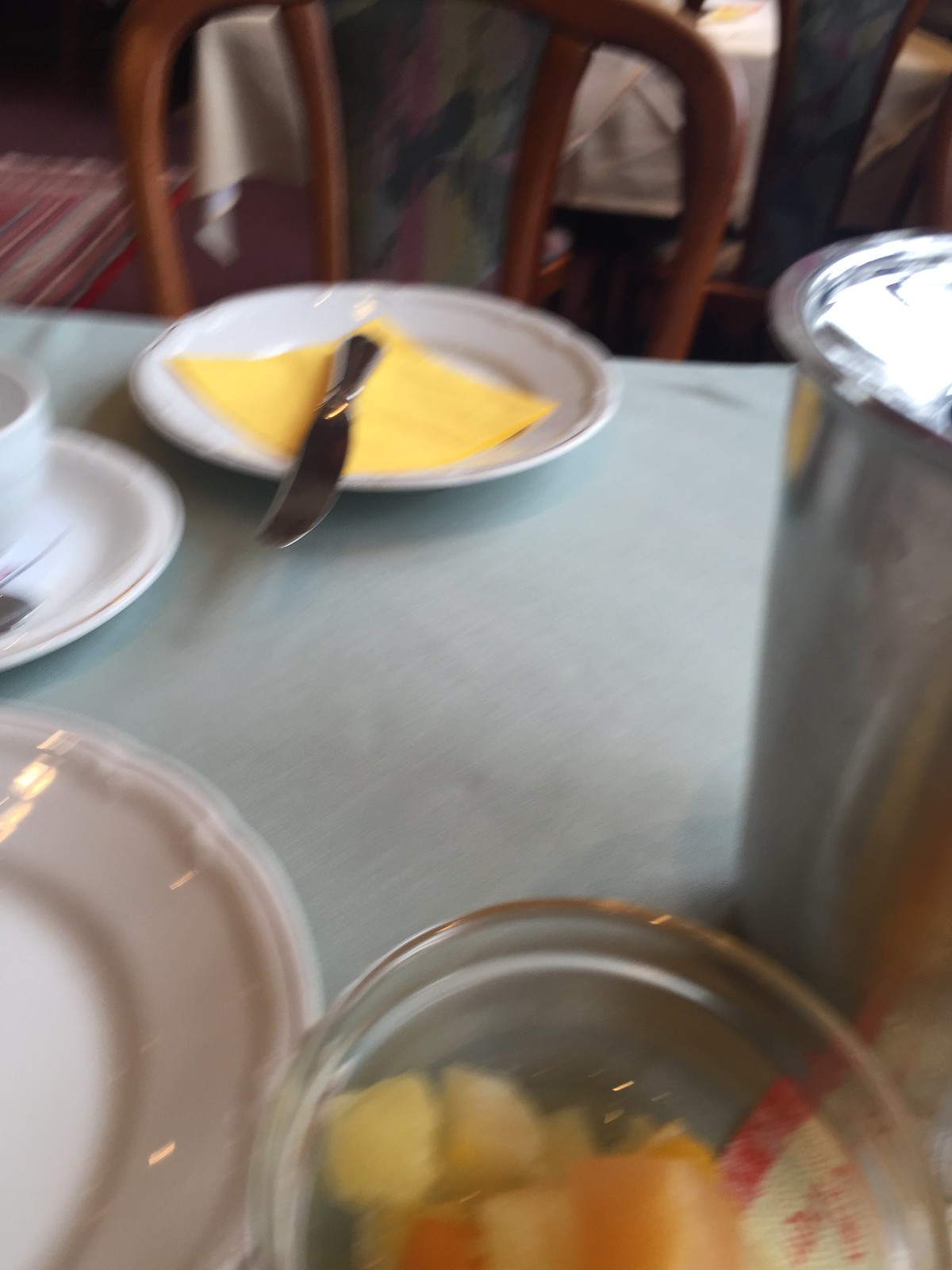This is a somewhat blurred photograph of a square table, likely in a hotel or diner, adorned with a gray tablecloth. Positioned prominently in the foreground, a tall silver carafe sits on the right side. The table is set with several white porcelain plates, one featuring a folded yellow napkin that resembles a slice of cheese, and a butter knife laid across it with the handle inward and blade outward. Adjacent to the plates, a clear glass bowl containing chopped fruit—possibly cantaloupe, pears, or pineapple—stands out. A wooden high-backed chair with a fabric strip in its middle is visible behind the table. On the left, a saucer partially conceals a cup, implying the presence of hot beverages. Additionally, another table with similar settings can be partly seen in the background, contributing to the cozy, inviting ambiance of the establishment.